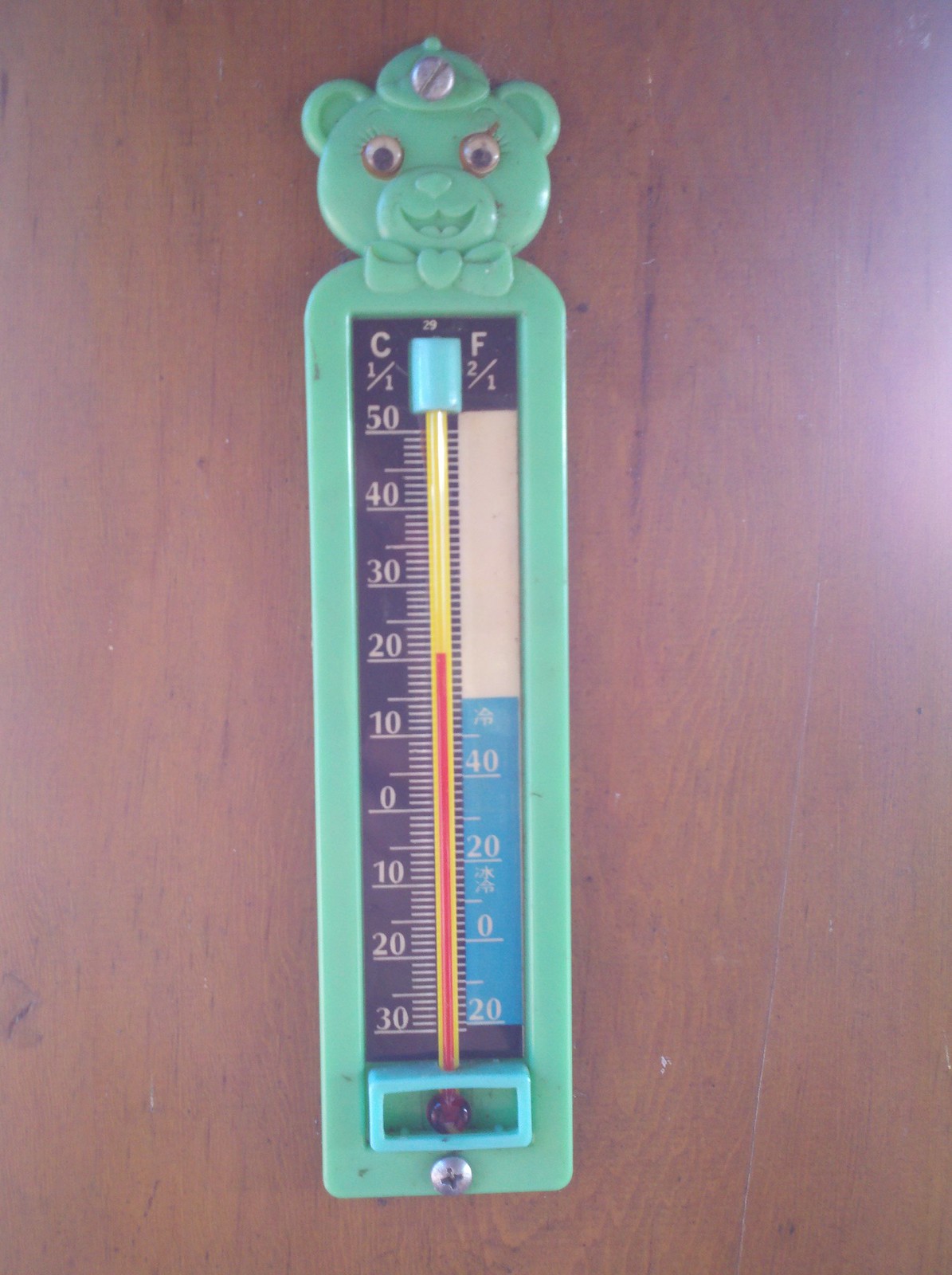The image depicts a downward view of a thermometer set against a dark brown background, likely a wooden table. The thermometer is framed by a turquoise blue casing. At the top of the thermometer, there is a bear face design featuring eyes with black pupils and white sclera, and a circular nose and mouth at the bottom. A single silver flat-head screw is positioned at the bear's forehead, suggesting that the thermometer could be mounted on a wall. At the bottom, another silver screw, this one a Phillips head, secures the structure.

The main body of the thermometer includes a turquoise rectangle with numerical readings on either side. On the left, the Celsius scale is marked in increments: 30, 20, 10, 0, 10, 20, 30, 40, 50 degrees, with 'C' at the top indicating Celsius. On the right, the Fahrenheit scale is displayed: 20, 0, 20, 40 degrees, on a blue background, with 'F' at the top indicating Fahrenheit.